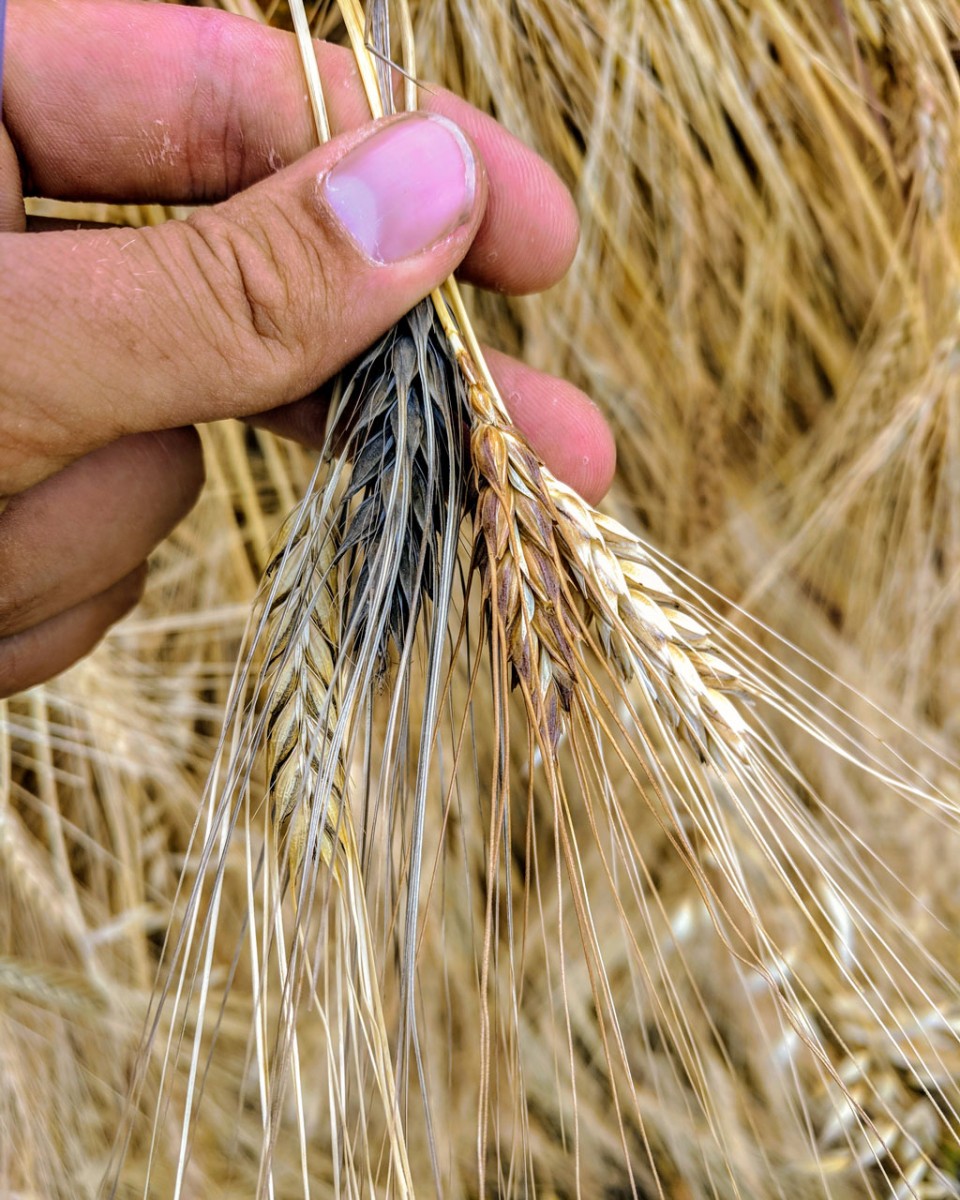A close-up photograph captures a hand holding a piece of hay, prominently featured in the upper left-hand corner of the image. The hand's index finger, middle finger, and thumb are extended, grasping the stem of the hay. The hay itself exhibits a mix of yellow hues with some blackish discoloration at its base before branching out. The blurred background showcases more hay, emphasizing the sharp focus on the hand and the single piece of hay being held.